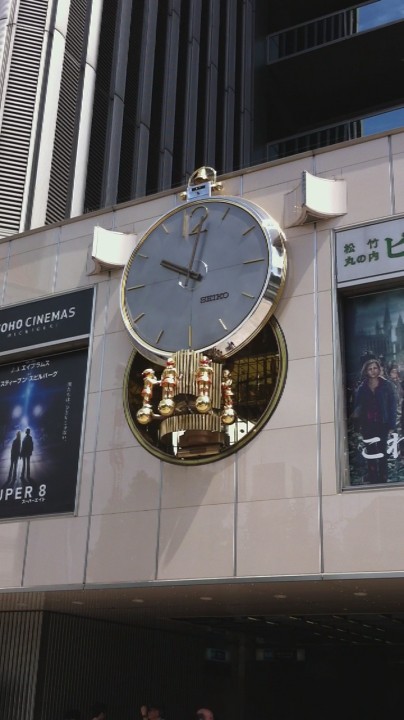The photograph captures a vertical image of an urban movie theater façade, distinguished by its square, tan-colored tiles with intersecting white lines. Central to the image is a striking clock mounted on this tiled wall. The clock is notable for its round face set within a shiny metal bezel, which resembles a giant stopwatch. Unlike conventional clocks, it bears the number '2' where the '12' would typically be, and the remaining hours are marked by silver lines. The clock's face is branded with 'Seiko' in black and features two black or silver hands, indicating the time is slightly past ten o'clock. Underneath the clock are intricate gold figures reminiscent of revolving clockwork mechanisms, adding an ornate touch. Flanking the clock are two movie posters with oriental characters: on the left, a partially visible poster with black background displays "Soho Cinemas" and "Super 8," alongside shadowy figures; on the right, another poster also adorned with Asian letters. In the background, the tiled wall continues, affirming it is part of a larger exterior building structure.